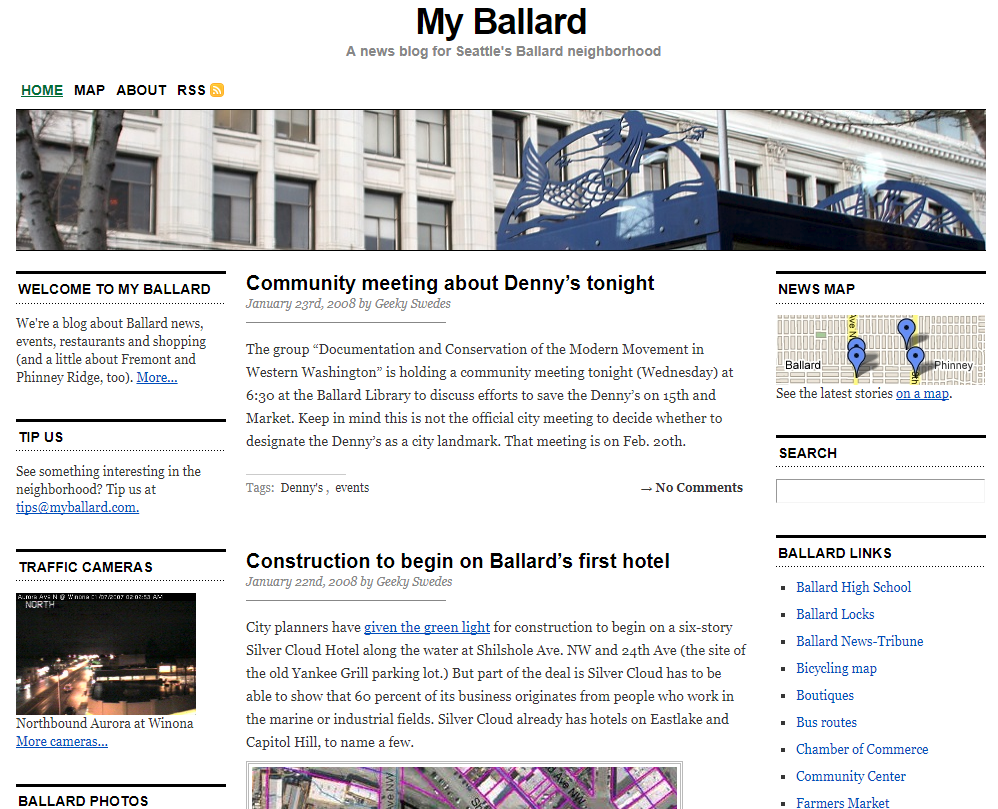**Caption: Seattle Ballard Neighborhood Blog Overview**

In the forefront of the image, a striking steel mermaid sculpture, turned sideways and finished in a weathered gray hue, crowns the entrance of a historic white stone building with multiple windows. This building, possibly an office or historical site, sets the scene for a detailed overview of a blog dedicated to the Seattle neighborhood of Ballard.

The blog, titled "Welcome to My Ballard," is a vibrant platform that covers local news, events, restaurant reviews, shopping spots, and occasionally includes content about nearby Fremont and Phinney Ridge. The homepage features a green, underlined "Home" link, along with an RSS feed icon represented by a small yellow square with white lines.

Highlighted in the blog is an announcement about a community meeting scheduled for Wednesday at 6:30 PM at the Ballard Library. This meeting, organized by the Documentation and Conservation of the Modern Movement in Western Washington, aims to discuss efforts to preserve the Denny's on 15th and Market. It notes that the official city meeting to consider designating the Denny's as a city landmark is set for February 20th.

Also displayed on the blog are various interactive elements, such as a news map showing the latest stories across the city and locations of traffic cameras. One of the significant updates mentions the commencement of construction on Ballard’s first hotel.

Dated January 22, 2008, and authored by the "Geeky Swedes," the blog aims to keep the community informed and engaged. It encourages readers to send tips and interesting observations to Tips@MyBallard.com. Additionally, the sidebar contains useful links to high schools, news outlets, bicycle maps, boutiques, bus routes, the Chamber of Commerce, community centers, and farmers markets.

This blog serves as a comprehensive resource for residents and visitors alike, reflecting the dynamic spirit of Ballard and its surrounding neighborhoods.